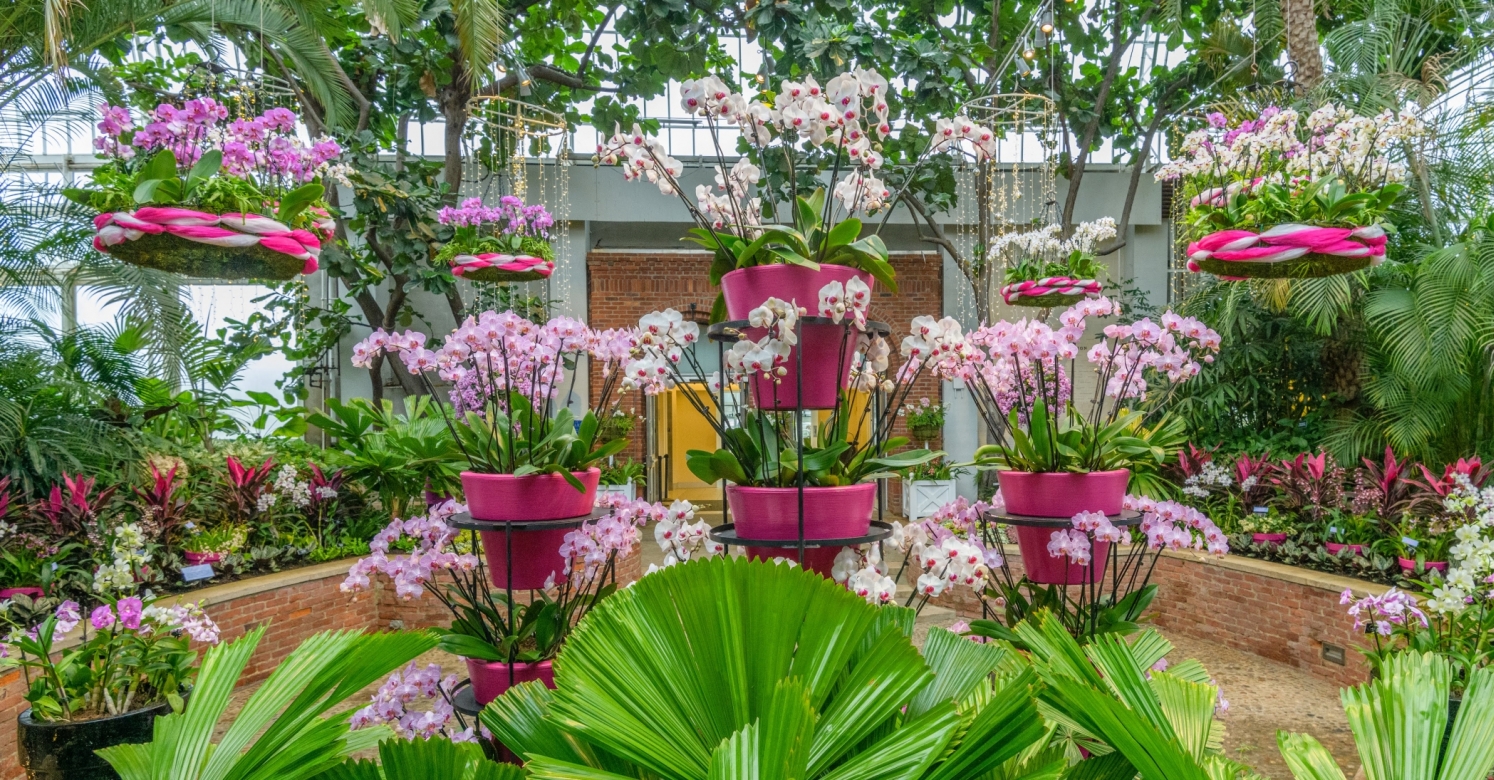The photograph captures the interior of a flower shop or nursery, characterized by an impressive display of colorful plants and flowers arranged in a symmetrical and aesthetic manner. The bottom section features fanned-out green leaves, creating a lush base. Moving upward, the middle section showcases several pink flower pots, all uniformly filled with vibrant flowers in hues of white, purple, and pink. Above these, hanging from the ceiling, are round, circular pots, similarly brimming with white, purple, and pink flowers, adding a vertical dimension to the arrangement.

To the sides, low brick walls form planters filled with an array of foliage and smaller plants, flanking the main floral display. In the background, a brick-and-mortar wall with windows and yellow doors adds to the charming ambiance. The symmetrical arrangement of plants and the meticulous color coordination make the scene both inviting and visually pleasing, epitomizing a beautifully curated plant store or nursery.